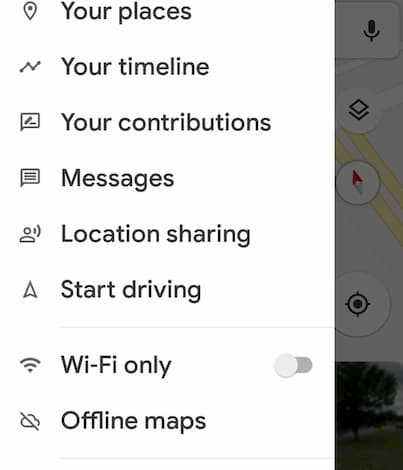This image is a screenshot capturing a menu overlay within a map application. To the right-hand side, partially visible in the background, is a street map characterized by gray shading with white and yellow road lines and a snippet of a street view picture. Dominating the image is a pop-up menu designed for filtering searches titled "Your Places." It features a pin icon, followed by a line graph icon with the label "Your Timeline," a speech bubble labeling "Your Contributions," and another speech bubble tagged "Messages." Further down, the menu lists "Location Sharing" next to an icon of a person speaking, an up arrow labeled "Start Driving," and a gray bar labeled "Wi-Fi Only" with a toggle switch currently set to off. The final option in the list is "Offline Maps," marked by a cloud icon with a line through it. The entire menu is presented on a white background, offering a comprehensive set of options for user interaction within the map application.